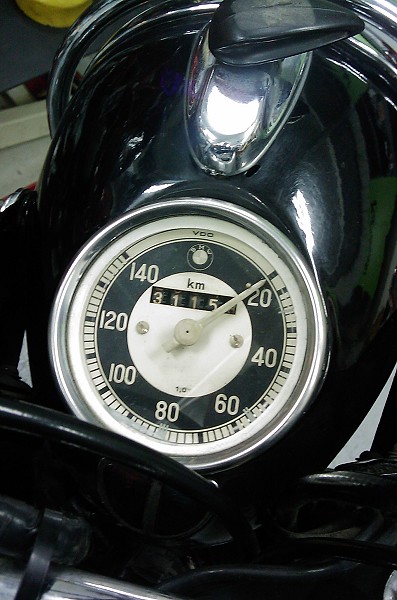The image captures the intricate details of a motorcycle's meter, prominently displaying the craftsmanship associated with a BMW model. The motorcycle features a sleek black frame with a glossy finish accentuated by silver accessories, creating a sophisticated and polished look. Overarching the meter is a silver bar that adds structural elegance and support.

At the center is the primary focus—a white circular meter embedded with the distinct BMW logo. The meter reads 3115 kilometers, with the "KM" designation clearly indicating the unit of measurement. The numeric values are spread in a semi-circle, expanding from 20 on the right, through increments of 20 (40, 60, 80, 100, 120), and culminating at 140 on the left. These numbers are rendered in white, contrasting sharply against the black segmented background. Intervals between the main numbers are marked by smaller lines, ensuring precision and easy readability.

The meter's needle is positioned at the bottom, suggesting that the motorcycle is currently stationary and the engine is not running. The overall composition and detailed elements of the image reflect both the aesthetic design and functional engineering of the BMW motorcycle, highlighting its blend of elegance and performance.